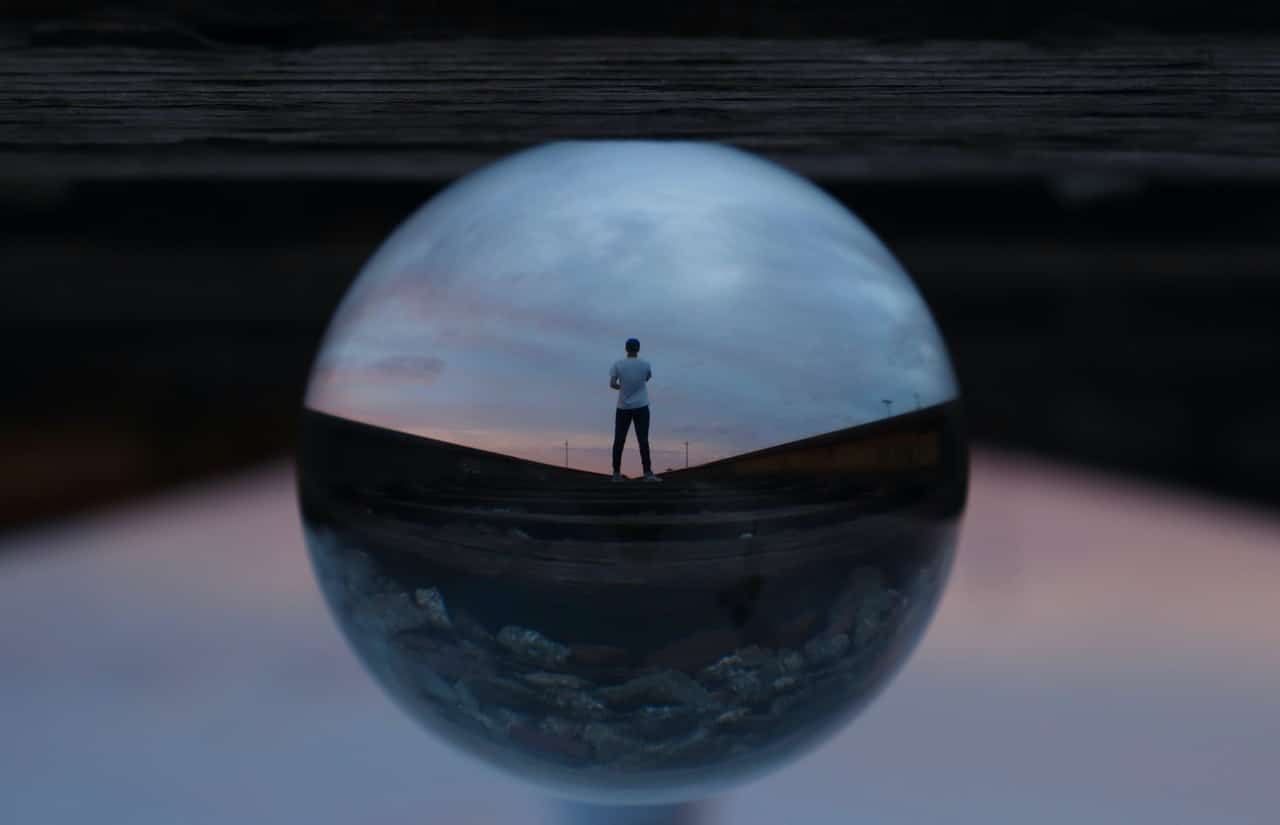The image depicts a surreal scene centered around a reflective orb placed on what appears to be a train track. The orb captures a detailed reflection of a man standing on the tracks, facing away from the viewer. He is dressed in a white shirt, black pants, and white shoes, and has short dark hair. In the reflection, the setting appears to be at dusk, with a sky bruised with hues of pink and gray clouds, allowing some blue to peek through. The background outside the orb shows a dark, almost water-like pattern with wood grain textures, blending with the colors of the sky reflected in the orb. The train track beneath the man is detailed, with visible stones between the wooden sleepers and metal rails. Dotting the horizon in the reflective image are several telephone poles, adding to the depth and realism of the scene. The overall composition of the image is dark at the top and lighter at the bottom, creating a stark and intriguing contrast.